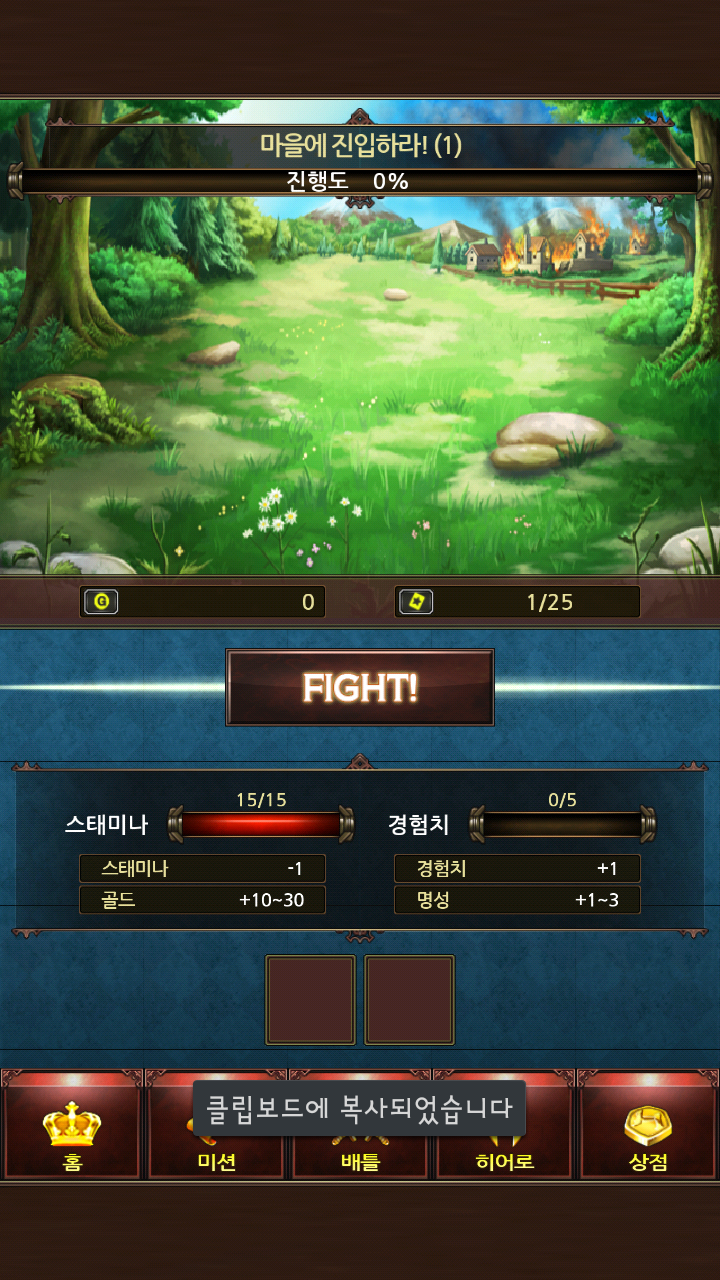Screenshot from a video game featuring an idyllic Asian countryside. The tranquil scenery includes soft rolling hills, smooth rocks, and a picturesque cottage. However, one of the cottages is dramatically ablaze, with flames contrasting against the serene environment. The sky is a clear, vibrant blue. Atop the screen, a banner with Asian characters is displayed. At the bottom, there's a brown box labeled "Fight" in white letters, followed by a series of Asian characters and numbers (e.g., +1, 1-3, 10-30). Additionally, gold images with red backdrops and more Asian characters are visible at the very bottom of the screenshot.